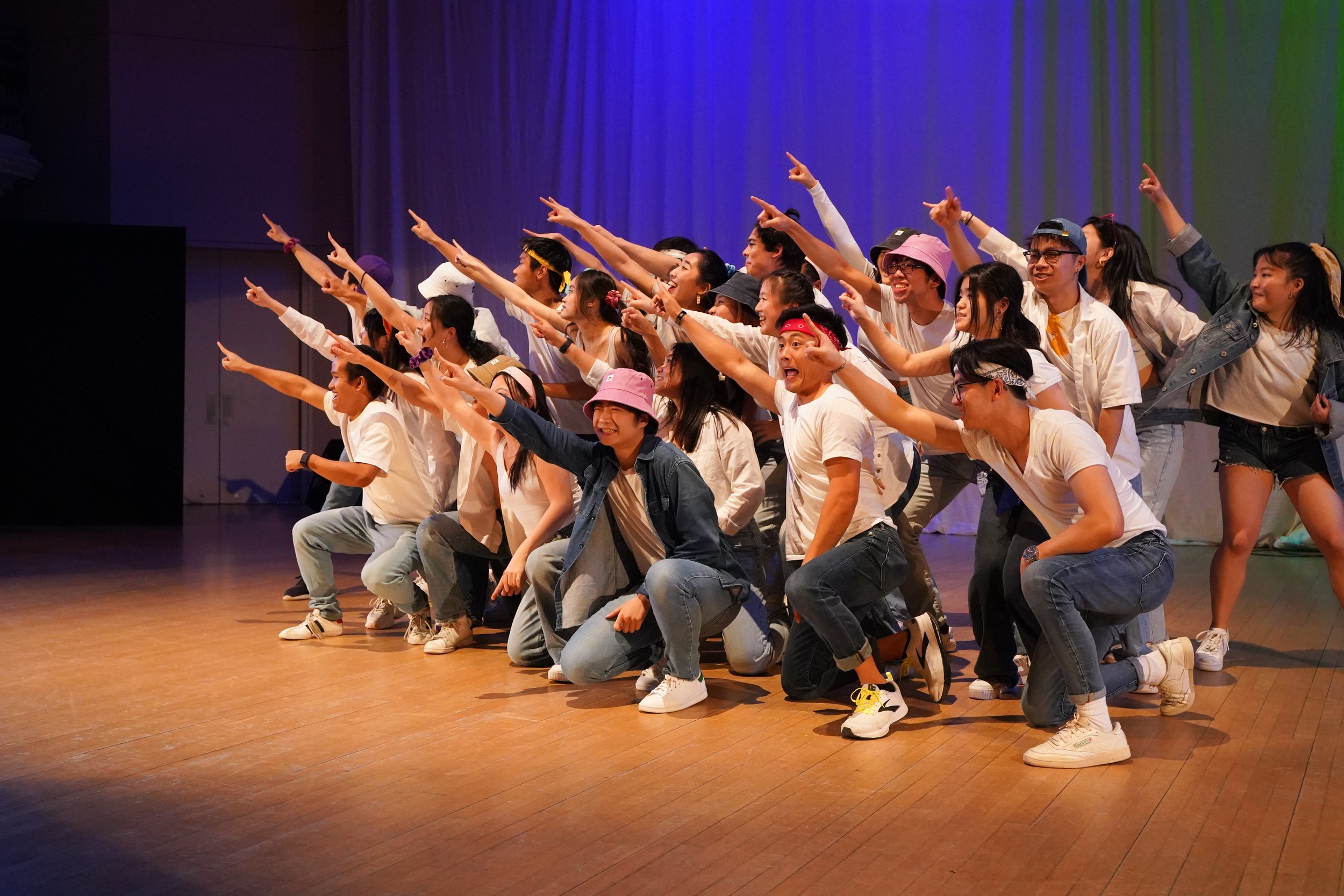In this captivating image, an Asian comedy troupe poses on a wooden theater stage, joyfully engaging with their audience. The ensemble, consisting of approximately 15 to 20 actors, extends their right arms outward in a unified gesture towards the crowd, their faces beaming with exuberant smiles. Much of the troupe's attire includes white shirts, complemented by denim jackets and jeans, with a few members donning shorts. A whimsical touch is added by several male actors sporting pink bucket hats. Almost all the actors wear white shoes, save for one individual positioned at the back. The backdrop is adorned with a silk screen that transitions from blue to green, creating a visually appealing gradient that enhances the overall scene. Stage left is discernible, indicating where the actors would typically make their exit. This lively tableau effectively captures the essence and camaraderie of the troupe, radiating a sense of happiness and connection with their audience.